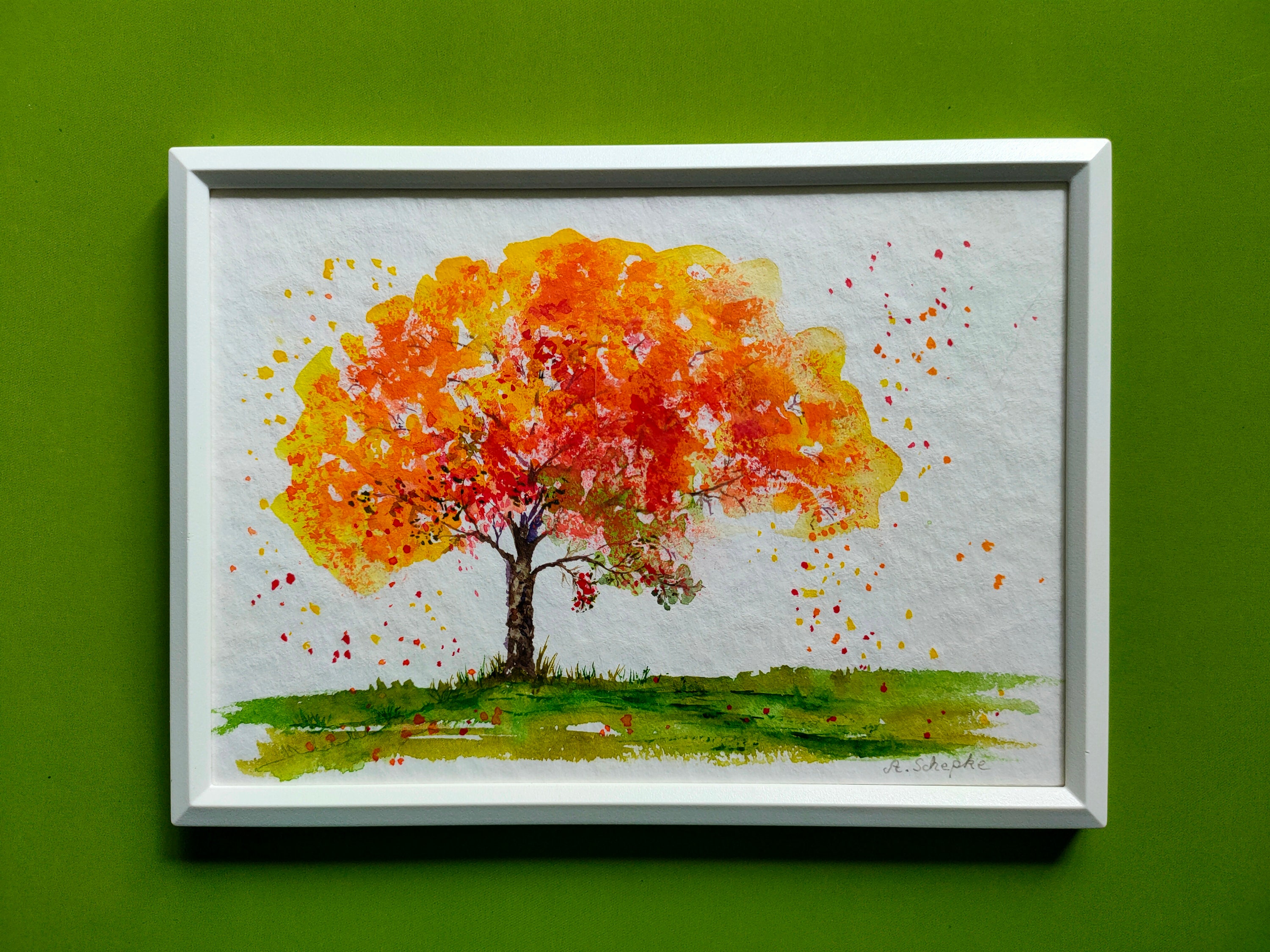The photograph captures a painting mounted on a pea green wall, encased in a white frame. The painting, which appears to be a watercolour on textured, slightly crinkled white paper, features a majestic, old tree with a thick, dark brown trunk standing in a field of green grass. The tree is adorned with vibrant autumn leaves in shades of red, orange, yellow, and some green, with additional dots in similar colors scattered around, giving the impression of leaves falling. The sky in the painting is left blank and white, setting a stark contrast to the colorful foliage. The bright autumn hues and fall embellishments create a vivid contrast against the green grass and the white space surrounding the scene extends to the edges of the frame. The whole composition suggests a distant perspective, showcasing the full grandeur of the tree and its seasonal transformation. The setting appears to be a gallery-like environment, as indicated by shadows cast by the frame on the wall and within the painting itself.